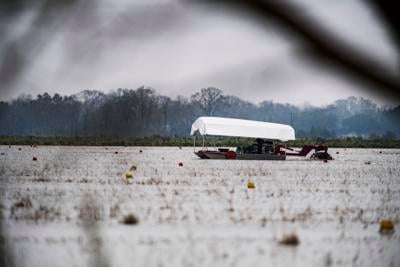This photograph depicts a serene wintry landscape characterized by a gray and white color palette. The scene features a snow-covered ground with patches of brown, dead grass poking through. In the foreground, blurry pieces of grass or ground cover suggest the photo was taken from a low angle, possibly through a plant or bush. The background reveals a line of barren trees, stripped of leaves, standing against the overcast gray sky.

In the middle distance, slightly to the right, there appears to be a body of water, possibly a flooded field that gives an impression of a farming landscape. Upon closer inspection, a wooden paddle boat equipped with a white canopy comes into focus. The boat, which looks like a two-pontoon type, has a paddle wheel at the back and is partially obscured by the surrounding elements, making intricate details hard to discern.

Adding to the complexity of the scene, a red metal plow with a white cover is visible further into the right side of the photograph, enhancing the wintry agricultural ambiance. The entire scene portrays a calm, outdoor winter tableau with a blend of natural and man-made elements, covered in the stark beauty of winter.